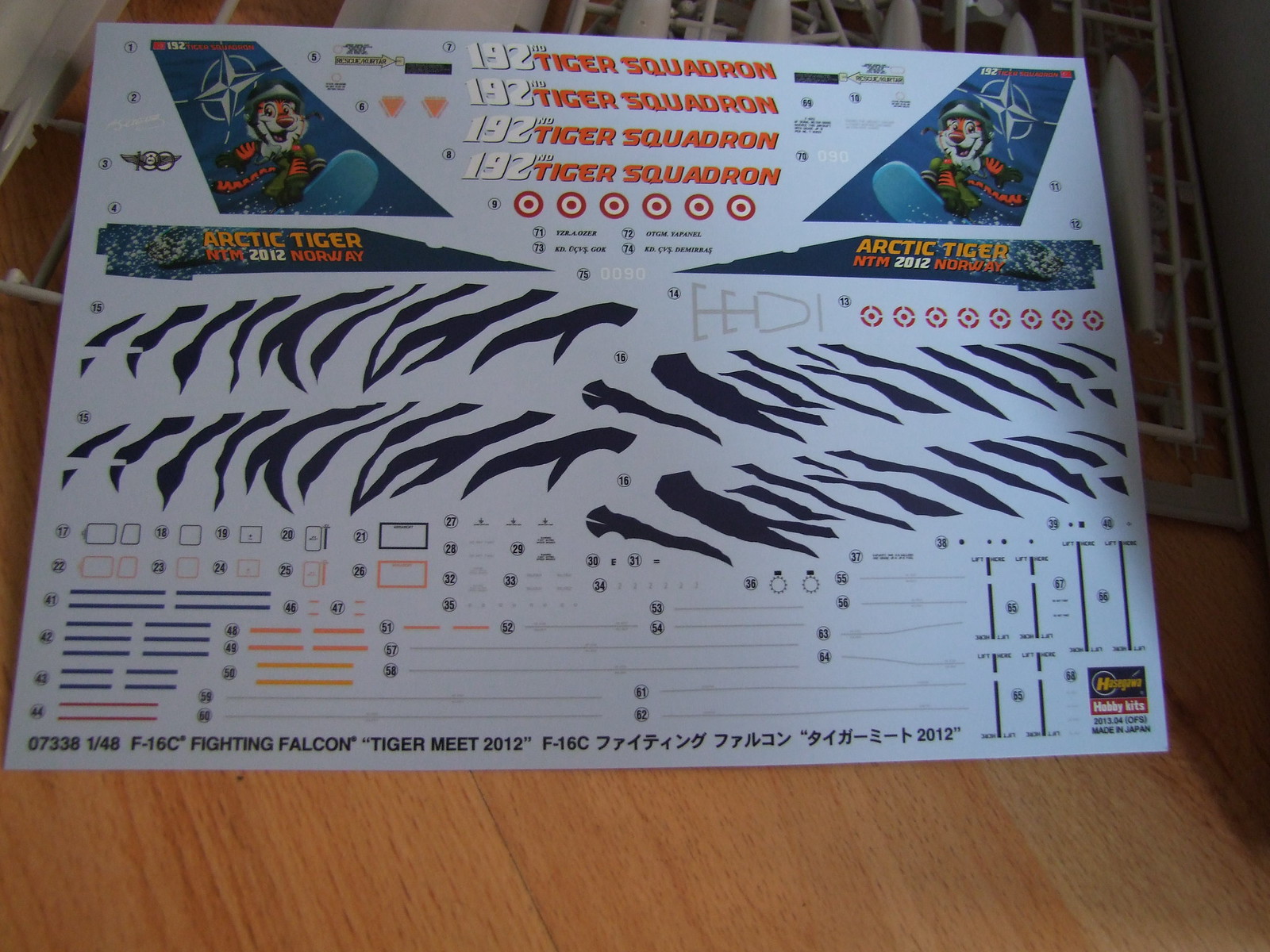On a wooden floor, there's a white sheet of paper filled with intricate details. Dominating the top left and top right corners, a cartoon tiger on a blue snowboard cheerfully smiles, wearing a helmet. This tiger image is repeated with a background icon resembling a northeast-southwest compass. The tiger features vivid orange and black stripes. Running down the center of the page, the phrase "192 Tiger Squadron" is prominently repeated four times. Below this, several red circles containing white circles and other red circles appear sporadically.

The bottom half of the sheet is dense with design elements: blackish streak markings, various tiger skin patterns, and several blank lines next to numbers, presumably for annotations. Additionally, the paper contains an assortment of colorful lines—blue, red, and orange—alongside rectangular and square boxes. At the very bottom, the text "Fighting Falcon Tiger Meet 2012 F-16C" and several footnotes are displayed, accompanied by writing in another language, likely Asian (Japanese or Chinese). The logo "Hasegawa Hobby Kids 2013.04 (05S) Made in Japan" is also found at the bottom right corner. The entire setup rests against a wall, with more items placed in the background, hinting at a bustling scene.